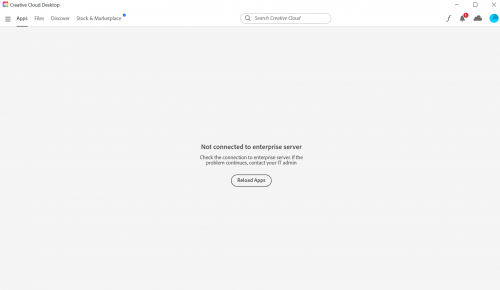This is a detailed screenshot of a desktop screen on a Windows computer. The primary application displayed is Adobe Creative Cloud Desktop. In the upper-left corner, the application title, "Creative Cloud Desktop," is displayed. Below the title, there is a navigation menu with options: "Apps," "Files," "Discover," and "Stock and Marketplace." Currently, the "Apps" section is selected, indicated by an underline.

To the right of the navigation menu, in the top-right corner, several icons are visible. A blue circle with a partial dark blue section, an icon resembling the letter 'S' or 'F,' a bell icon with a red notification dot, a cloud icon, and another blue circle follow the search bar, which currently displays the placeholder text "Search Creative Cloud". 

Alongside these elements, the generic window control buttons are present: a minimize button ('-'), a maximize/restore button (square), and a close button ('X').

In the center of the screen, a prominent message reads: "Not connected to enterprise server. Check the connection to the server. If the problem continues contact your advisor." Below this message is a "Reload App" button, likely intended to attempt reconnection or refresh the application.